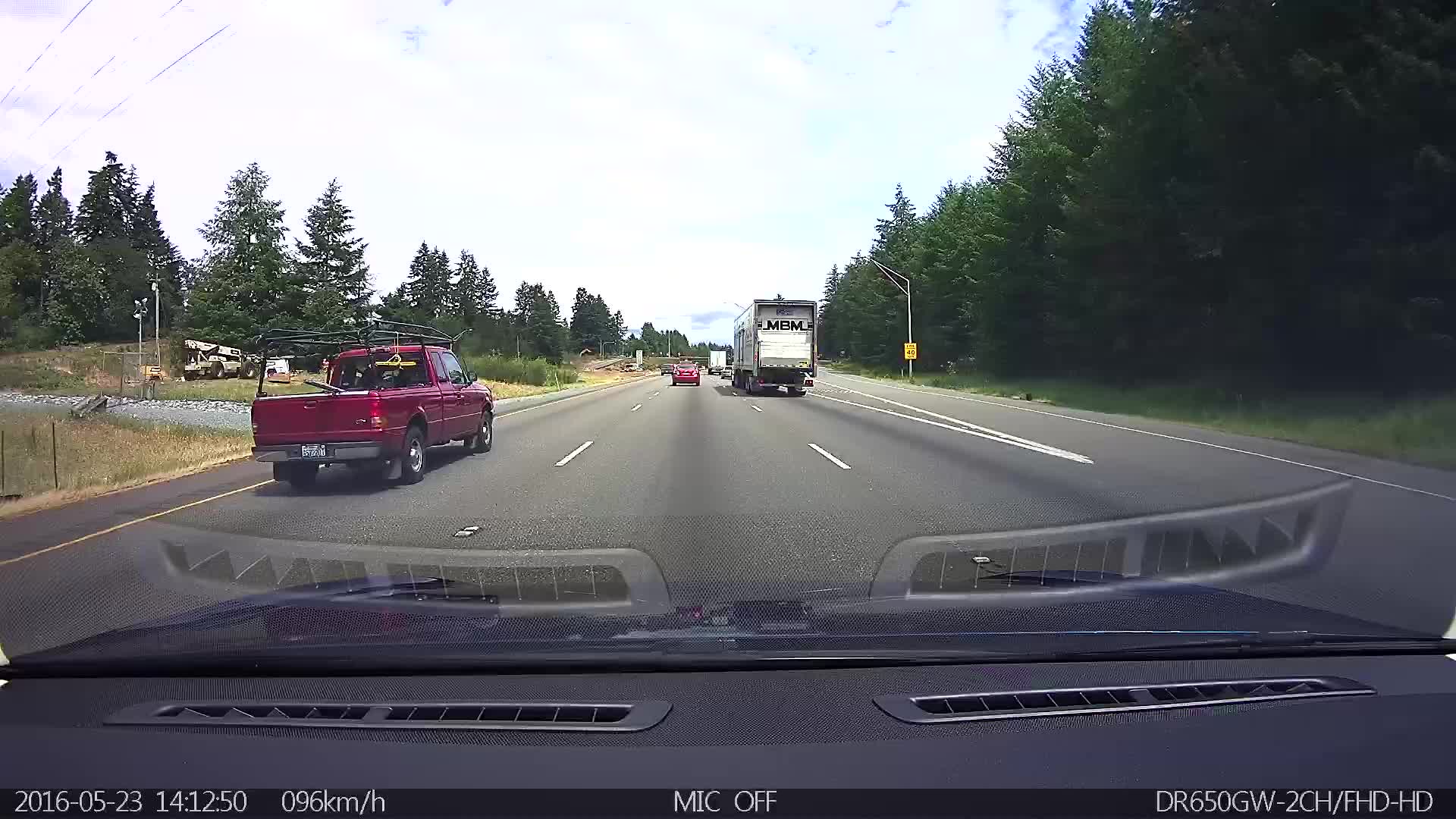In the foreground, a well-worn pathway forks into two directions, with one leading to the left and the other veering sharply to the far right. On the left side of the image, a cluster of mature trees stands tall, their leaves partially shading patches of dry grass below. Further in the background, another stretch of trees and grass can be seen, giving the scene a lush, yet somewhat sparse, atmosphere.

Dominating the left side, a vivid red truck is conspicuously parked, contrasting starkly with the natural surroundings. Toward the right, another truck is parked alongside additional vehicles that extend into the distance. The meticulously laid-out pathways are demarcated by distinct dash marks, effectively dividing the lanes.

Amidst this arrangement, a solitary black basketball lies inconspicuously yet poignantly in the backdrop, hinting at recent human activity. Encircling the entire scene is a two-layered fence, providing an enclosed yet accessible feel to the area. This comprehensive snapshot was originally intended for an Inside Dashboard ticket scenario.